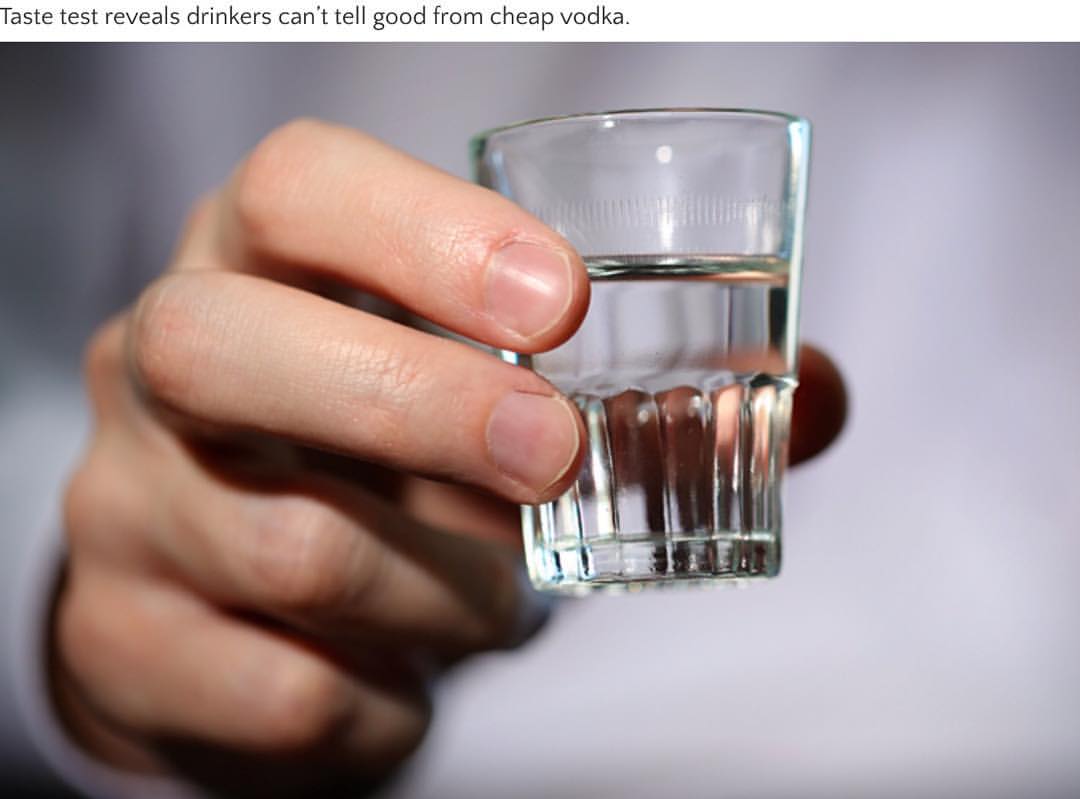The photograph, appearing to be from a newspaper or article, has a caption at the top that reads, "Taste test reveals drinkers can't tell good from cheap vodka." The image focuses on a person's hand of European descent, with a bare complexion and manicured fingernails. The hand, showing the thumb, index, and ring fingers, is holding a shot glass that contains a clear liquid presumed to be vodka. The shot glass has intricate designs at the bottom, getting whiter towards the top, and features curved ridges that run down its halfway portion. The background reveals the person's shirt, which is white but appears out of focus.